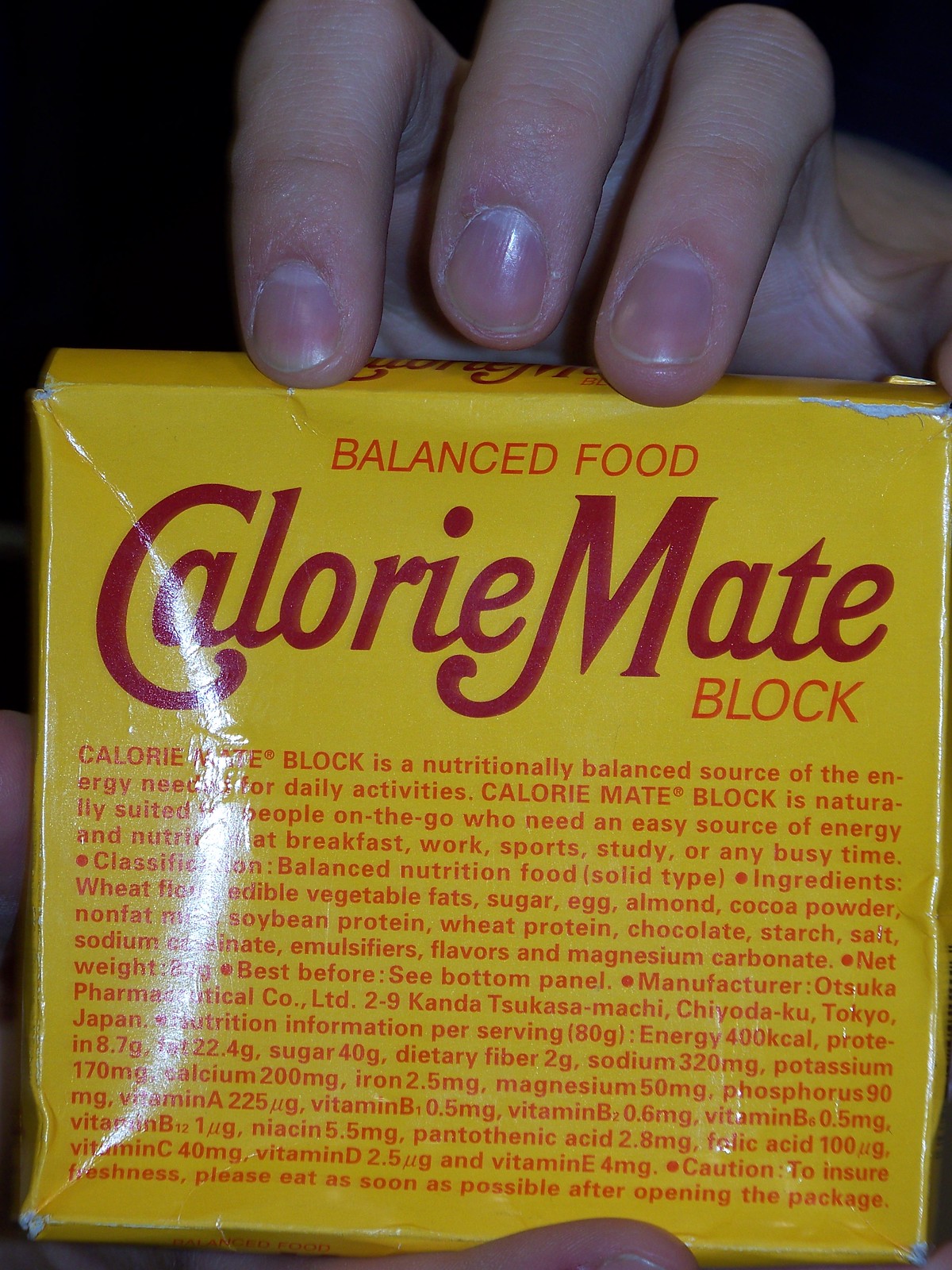In the image, a hand delicately holds a vibrant yellow box, prominently labeled "Balanced Food Calorie Mate Block." The text on the box specifies that "Calorie Mate Block is a nutritionally balanced source of the energy needed for daily activities." Additional writing on the packaging explains its suitability for busy individuals seeking an easy source of energy and nutrition during breakfast, work, sports, study, or other demanding times. The product classification mentioned is balanced nutrition food in solid form. Ingredients listed include wheat flour, edible vegetable fats, sugar, egg, almond, cocoa powder, nonfat soybean protein, wheat protein, chocolate, starch, salt, sodium carbonate, emulsifiers, flavors, and magnesium carbonate. Due to a glare in the photo, the net weight is obscured, though it indicates the best-before date is on the bottom panel. The hand grasping the box reveals three fingers resting atop the package and a partial view of a thumb beneath it.